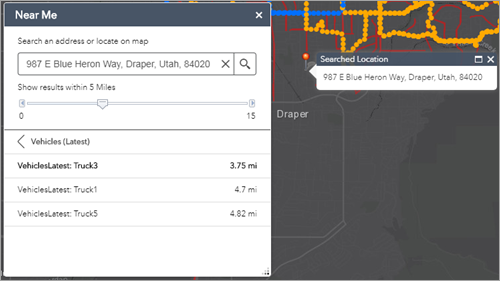Screenshot of a Vehicle Tracking Mapping Application

In this detailed screenshot of a mapping application, we observe a gray sidebar on the left labeled "Near Me," indicating a search function for nearby locations. An address has been entered into the address bar: "987 East Blue Heron Way, Draper, Utah, 84020." To the right of the address bar, there is an 'X' button for canceling the entered address and a magnifying glass icon indicating a search.

The application displays real-time locations of various vehicles. Specifically, it shows that "Truck 3" is 3.75 miles away, "Truck 1" is 4.7 miles away, and "Truck 5" is 4.82 miles away from the searched address. These vehicle statuses are updated under the "Vehicles Latest" section.

The interactive map itself features several colored dots—orange and blue—and red lines providing a visual representation of routes and locations. A pin labeled "Search Location" marks the specified address on the map.

This detailed visualization aids in tracking and managing vehicle locations with precision in Draper, Utah.